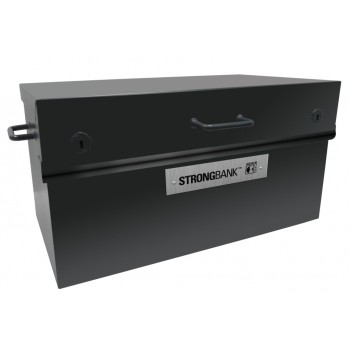The image depicts a decently large rectangular black toolbox, prominently positioned and nearly filling the entirely white background. The toolbox is angled diagonally with the left side closer to the viewer. It features two levels with the taller lower level bearing a silver plaque inscribed with "Strong Bank" in black letters. This sturdy box has a metallic silver handle on the top part, accompanied by two keyholes or locks positioned to the right and left of the handle. Additionally, a handle extends from the top left side of the toolbox, enhancing its functionality. The combination of black, gray, and silver hues, along with the clean, solid white background, suggest the image is likely intended for a product listing, emphasizing its robust and secure design for potential buyers.